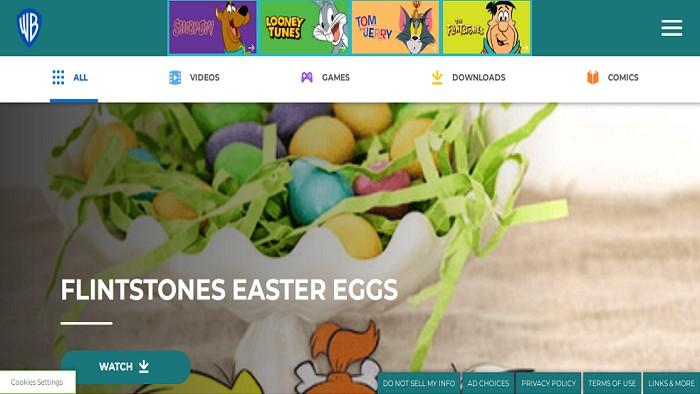The webpage displayed is dedicated to Warner Brothers Animation. The top header features a banner with rectangular images displaying well-known cartoon characters and titles such as Scooby-Doo, Looney Tunes, Tom and Jerry, and The Flintstones. Below this banner, there’s a navigation menu with options labeled "All," "Video," "Games," "Downloads," and "Comics." Each menu option is accompanied by a colored icon—blue, purple, yellow, and orange, respectively.

A prominent header image showcases a decorative bowl filled with crepe paper and dyed Easter eggs, labeled "Flintstones Easter Eggs." Below this header, there is a button prompting users to "Watch." 

At the very bottom of the page, users will find various settings and policy options. A white button with black text allows users to configure "Cookie Settings." Additionally, there are teal boxes with white text for options such as "Do Not Sell My Info," "Ad Choices," "Privacy Policy," "Terms of Use," and more. 

Notably, at the footer of the Flintstones Easter eggs header image, the top parts of the cartoon characters Bam Bam and Pebbles are partially visible, though they are mostly cut off.